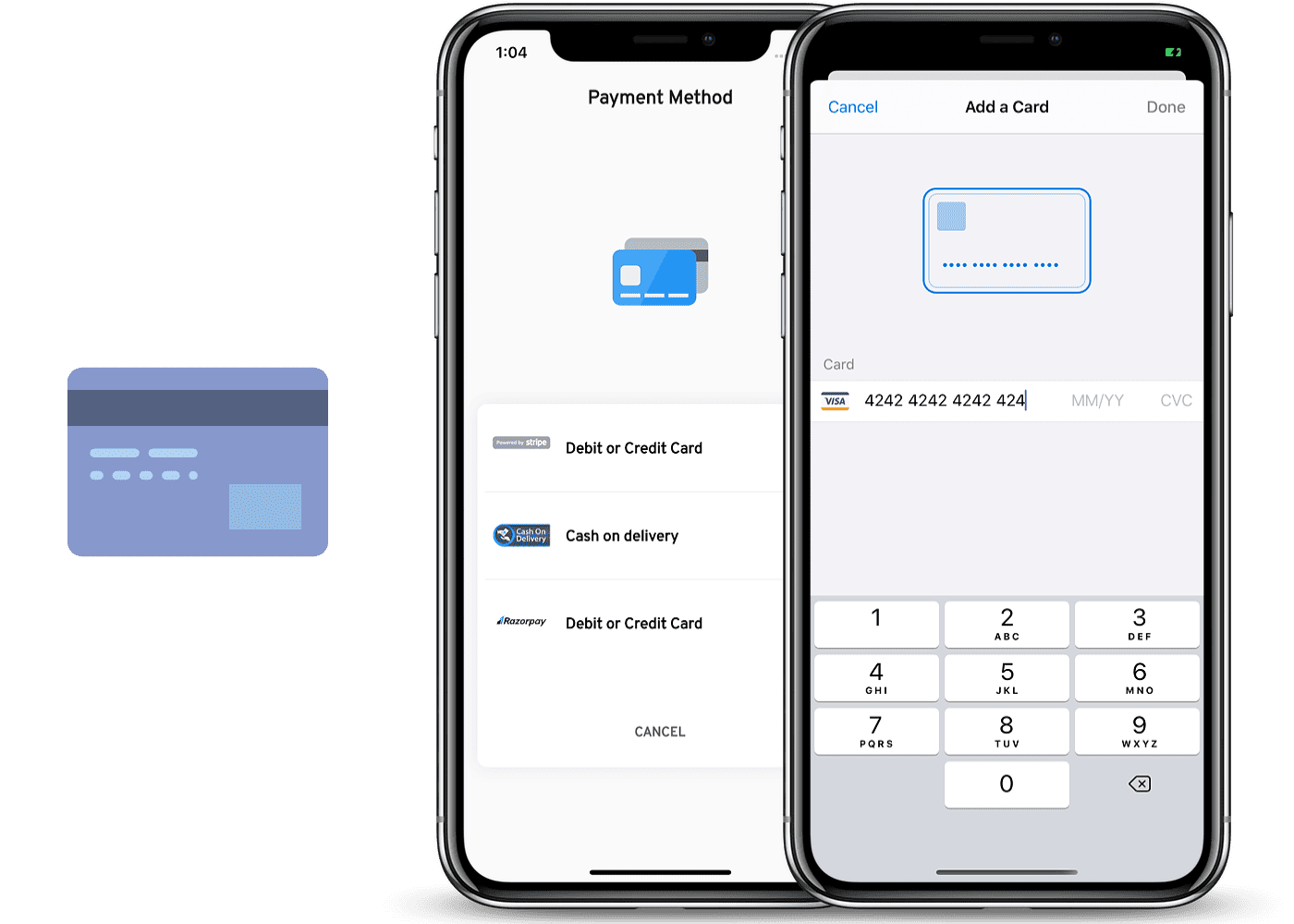The image displays a smartphone screen featuring a user interface for adding a credit card as a payment method. The interface is primarily white with black text and is depicted on a smartphone with silver borders. The top section of the screen shows "Payment Method" at the top and displays the back of a blue credit card. Below this heading are various payment options: "Debit or Credit," "Cash on Delivery," and "Debit or Credit through Razorpay."

A cancel button is also present in the interface. The second part of the screen shows another smartphone interface, prominently featuring a blue "Cancel" button, a central "Add a Card" button, and a "Done" option. This screen also displays the back of a credit card, specifically a Visa card with the number 4242 4242 4242 4242. Below the card image is a virtual keyboard for entering additional card details such as expiration month, year, and CVC.

The image serves as an instructional guide, demonstrating to users how to add a credit card or other payment methods on their smartphones. The background is predominantly white, highlighting the different screens and steps involved in the process.